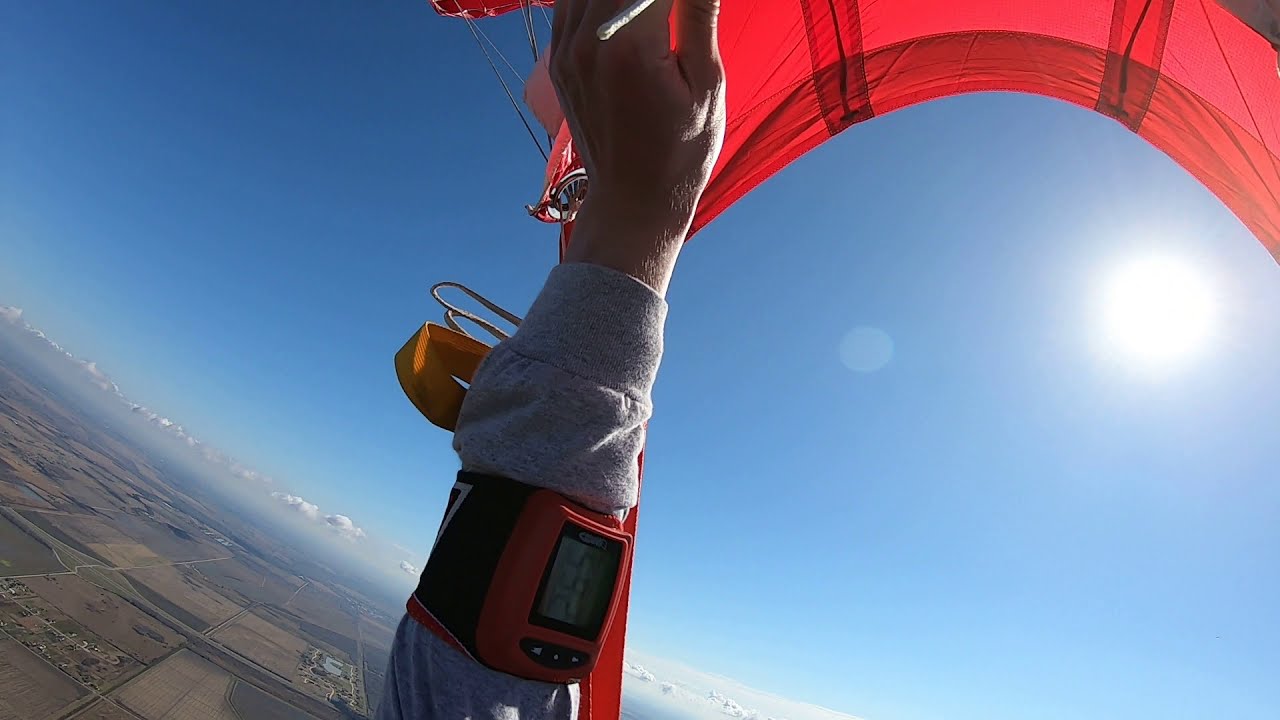The image captures a thrilling point-of-view shot of someone paragliding high in the sky. The red parachute above is fully extended, with black and gray wiring extending down toward the handles the person is gripping. The focus is on the person's left arm, clad in a gray sweatshirt, with a meter displaying the number 592 strapped on the forearm. Below, a patchwork of farm fields, distant roads, and tiny houses are visible, giving a bird’s-eye view of the sprawling landscape. Most of the clouds are situated below the paraglider, enhancing the sense of altitude. The sun is prominently visible on the center right of the image, illuminating the blue sky and casting a breathtaking view of the land below.